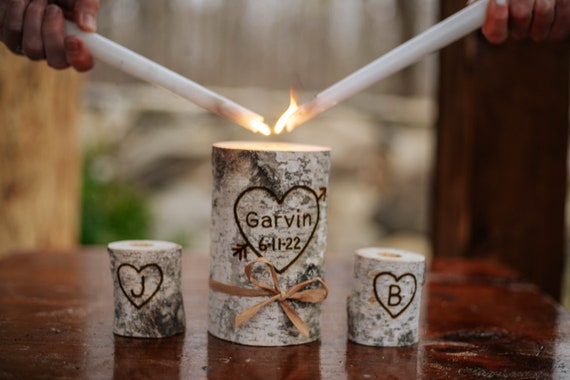The image depicts an outdoor scene with a glossy brown wooden table as its focal point. On the table, three candles are arranged, with a larger candle flanked by two smaller ones. The central, largest candle bears the name "Garvin" and the date "6-11-22" inside a heart, suggesting a couple’s wedding date. This large candle is adorned with a brown ribbon at its base. To the left of it, a smaller candle features the letter "J" encased in a heart, while the smaller candle to the right displays the letter "B" similarly encased. From the top of the image, two hands, each holding a long white candle, are collaboratively lighting the larger central candle, creating a shared moment of unity.